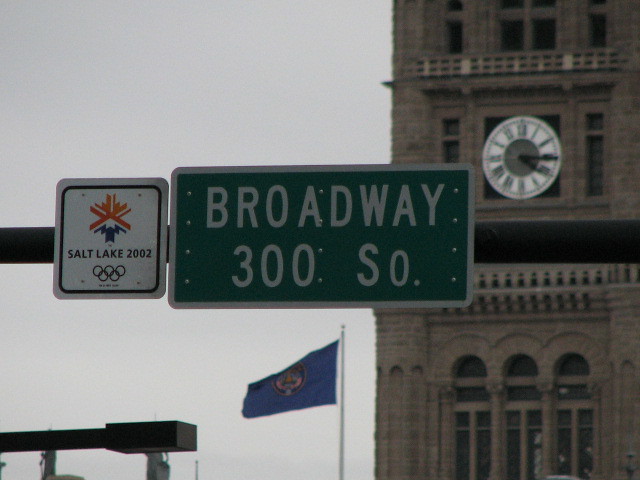The photograph is set outdoors under a sky that alternates between blue and gray due to cloud cover. Dominating the right side of the image is a tall, multi-story building made of grayish-brown brick, featuring arched windows and a prominent white clock face with black Roman numerals and thick black hands, situated at its center. Adjacent to this building is a flagpole flying a blue flag adorned with an emblem, extending leftward in the image. In the foreground, a street sign mounted on a horizontal black bar reads "Broadway 300 South" in green with white text. Below it, a rectangular white sign with a red and blue emblem commemorates the Salt Lake City 2002 Olympics, showcasing the Olympic rings and torch. Beneath these signs is a modern streetlight, constructed from black metal. The picture captures an intricate blend of historical and modern elements against a backdrop of varying sky tones.